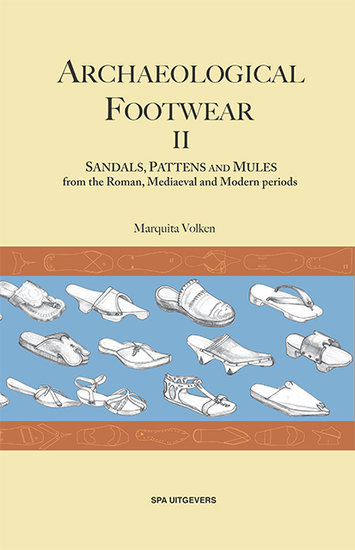The image displays a book cover with a rectangular orientation. The background is predominantly a tan or light brown color. At the top, in black letters, it reads "Archeological Footwear II," followed by the title "Sandals, Patterns, and Mules from the Roman, Medieval, and Modern Periods" authored by Marquita Vulcan. This header section features two black horizontal lines for separation.

Midway down the cover, there is a rust-colored banner adorned with various shoe prints, below which a large blue area showcases white drawings of different types of sandals and mules. The rust-colored banner with shoe prints reappears near the bottom. Finally, at the bottom in black letters, it says "Spa, Up-Givers."